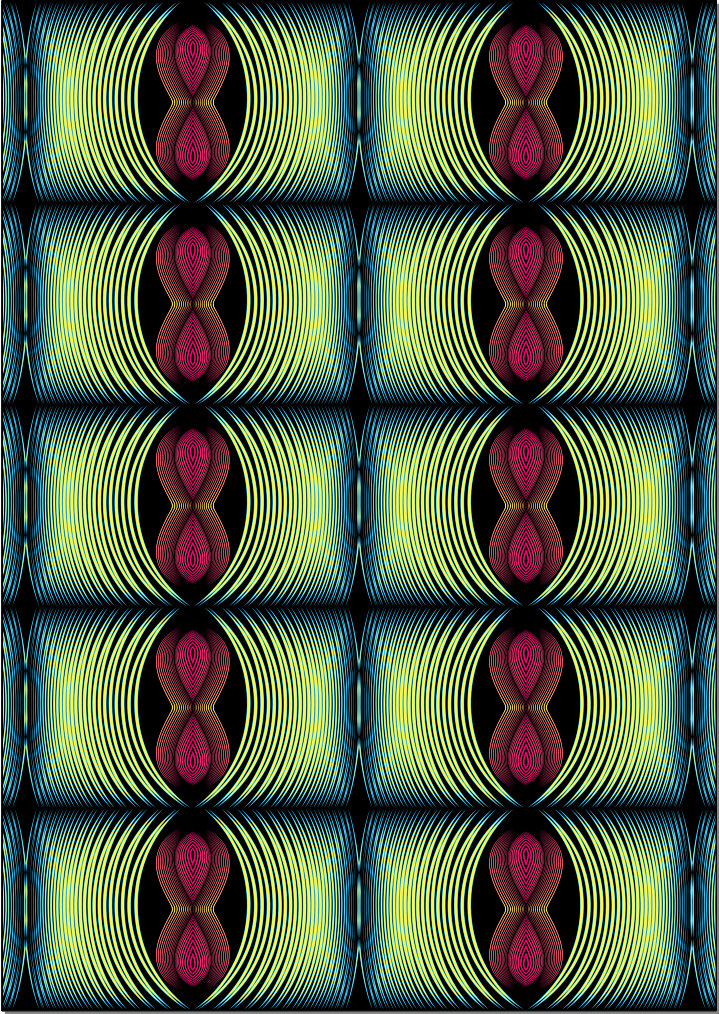This graphic image features a pattern of 10 horizontally oriented, rectangular figures. Each rectangle showcases a design predominantly using colors such as blue, yellow, red, magenta, brown, and black. Central to each rectangle is an eye-shaped or hourglass-like figure, evocative of a figure 8. This central motif is rendered in shades of red and brown with a hint of magenta or pink, set against a black background. A thin gold or arc-like yellow line accentuates the waist of the figure, radiating outward to the edges of each rectangle. The repetitive pattern extends seamlessly to the left and right, linking additional rectangles featuring blue elements. The overall impression is a mesmerizing, wavy sequence of interconnected figures, visually unified by their almost hypnotic, swirling designs.